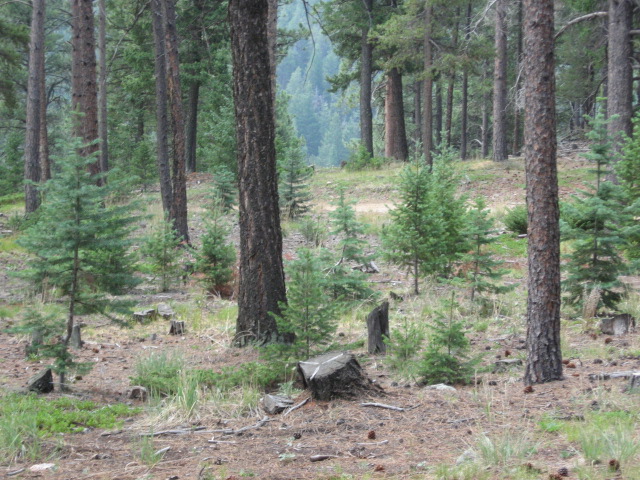The image captures a serene, higher-elevation forested mountainside, characterized by a mix of mature and young fir trees. The area appears to be an open, logged, and replanted clearing, evidenced by tree stumps scattered across the brown, needle-covered forest floor with minimal underbrush. Small fir saplings, not exhibiting the long needles typical of pines, dot the landscape, some standing about five feet tall. Amongst them, mature tree trunks rise, nicely spaced, occasionally showing signs of old fire damage. The sparsely populated clearing allows an unobstructed view across the valley, where thicker forested areas extend into the distance. The lighting suggests early morning, adding a tranquil atmosphere to the rejuvenating, rolling terrain.